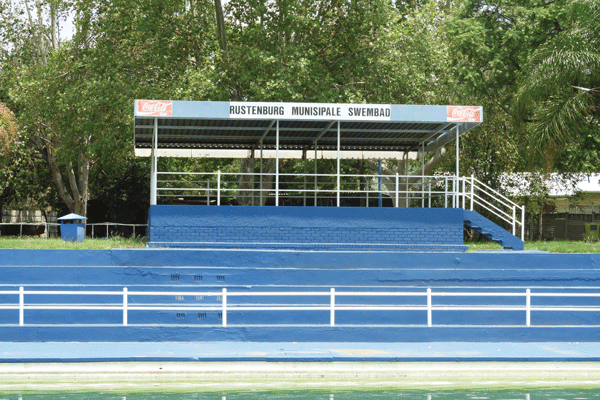This photograph, taken in an outdoor setting, captures what appears to be a racecourse or track area, likely used for events or spectating. At the bottom of the image, there is a green path followed by a blue sidewalk. A light blue wall with white stone fencing rises above these, with several additional blue walls layered higher up. The foreground features a blue and white platform which includes a shaded seating area, presumably for viewers. Adding to the official look, the platform prominently displays red Coca-Cola logos and the text "Rustenburg Municipal Swim Bad" in black lettering. This platform also includes a blue staircase on the right side, which appears to provide access for spectators. Beyond the platform, the background reveals a grassy area, trees, some wooden fencing, and distant buildings, contributing to the serene atmosphere. Notably, a blue trash can and a recycling bin are positioned to the left. The bright colors and structured design suggest a well-maintained public facility.